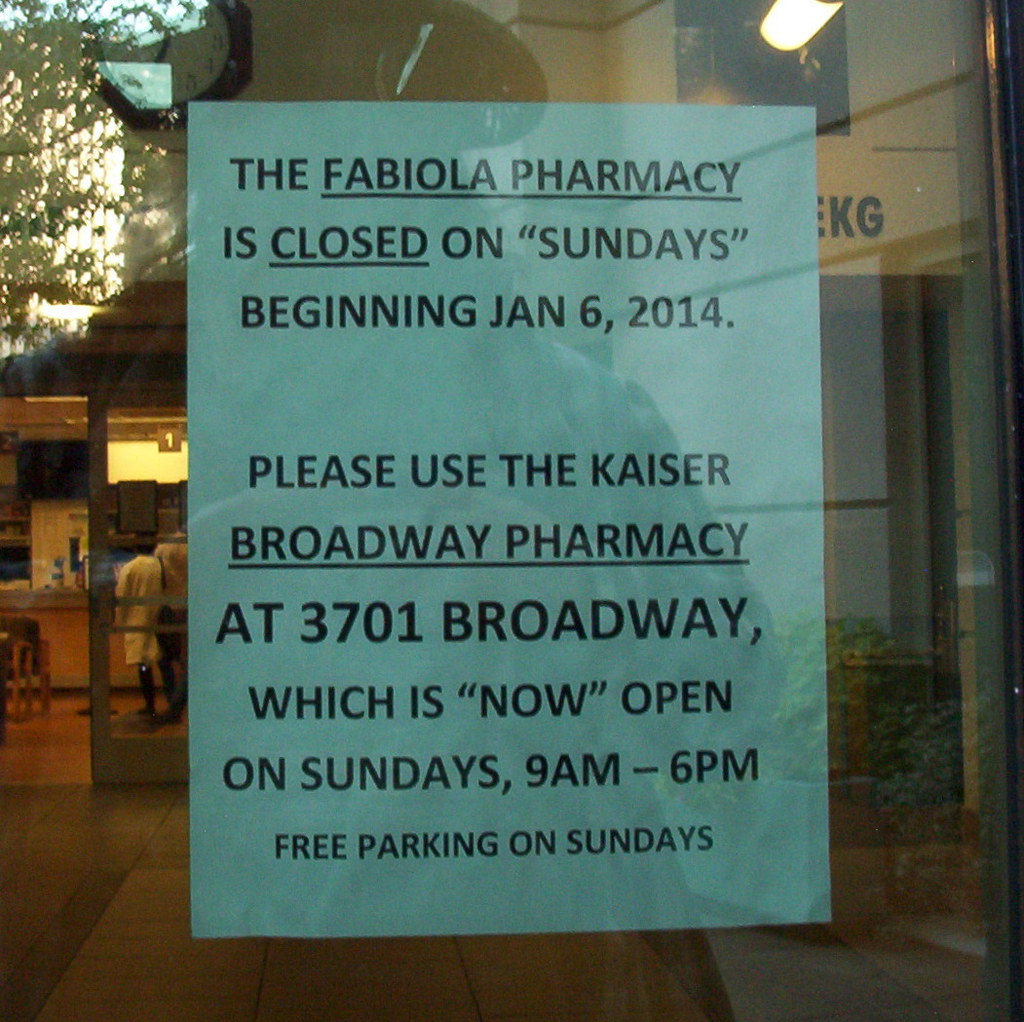This photograph captures a blue sign with black text, taped to the window of a commercial building, likely a pharmacy or hospital. The sign reads: "The Fabiola Pharmacy is closed on Sundays (beginning January 6, 2014). Please use the Kaiser Broadway Pharmacy at 3701 Broadway, which is now open on Sundays, 9 a.m. to 6 p.m. Free parking on Sundays." The text is entirely in capital letters. Reflections in the glass reveal the shadow of the photographer, a tree, and some bushes in the upper left corner. Inside the building, a number "1" is visible above people who appear to be standing in line, possibly at a pharmacy counter.